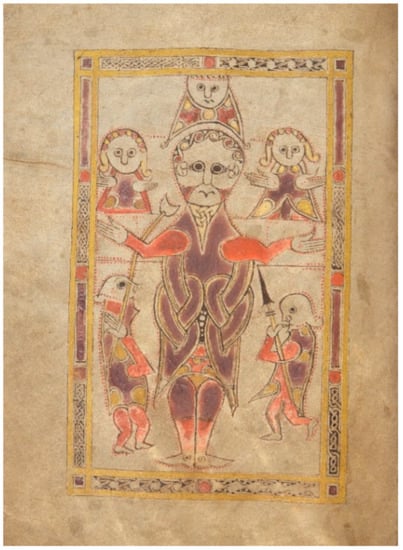This is a detailed photograph of an old medieval drawing, likely imprinted on a parchment-like material with a light cream to beige background. The artwork features a central figure who appears to be a king or a father, wearing an intricate, possibly orange or purple, robe draping down to the knees. The figure's arms are outstretched in a gesture of embracing, and atop his head sits a boy, with two females positioned on either side of him. Flanking the main figure at the bottom are two guards or attendants, each in orange outfits and wielding spears pointed upwards. Surrounding this central figure are a total of five individuals, some of whom could be angels with their hands outstretched, adding a mystical or religious aspect to the scene. The detailed colors include yellow, brown, maroon, and pinkish-orange, contributing to a rich, ancient aesthetic reminiscent of medieval hieroglyphics or manuscript illustrations.